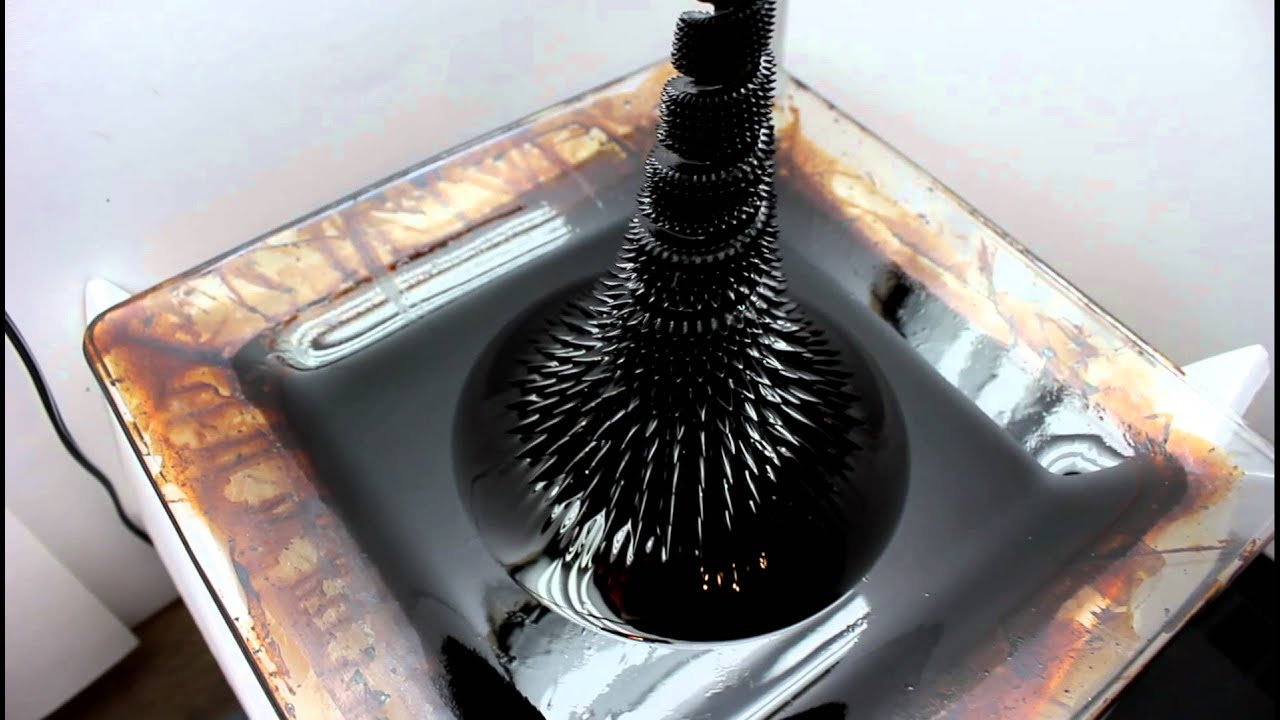In this intriguing photo, the backdrop features a mostly gray hue with subtle hints of purple and pink. Central to the composition is what appears to be a square, glazed ceramic dish, evocative of an old-fashioned ashtray. This dish, mottled with variegated shades of brown, tan, and amber, adds an element of rustic charm. At the dish's core lies a dark gray area, bearing a glossy black substance that suggests liquid metal or black ink. 

Emerging starkly from this dark center is a formidable object, resembling an intricately designed, spiked stand or brush. This object has a thick, rounded base from which numerous short, thin, sharp spikes radiate in all directions. The spikes extend up the stem, twisting and wrapping around it, lending the piece a dynamic, almost menacing appearance. The object’s surface is intensely glossy, reflecting light in a way that underscores its mysterious, polished nature.

The image also faintly depicts a blurred background with white walls and hints of a power cord descending down, adding a touch of mundane reality to this otherwise enigmatic scene. The reflection on the glossy surface of the dish subtly captures elements of its surroundings, enhancing the sense of depth and realism in the artwork.